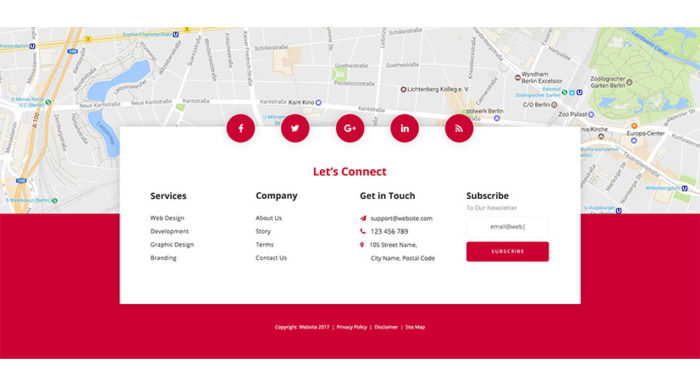The image is a split-screen design with the upper section displaying a detailed map adorned with various roadways, differentiated by shades of gray for roads, green for land, and blue for water bodies. Overlaying the top and bottom halves is a prominent white rectangular banner. 

At the top center of this white overlay, there are five circular red icons, each representing different social media platforms: a Facebook icon with a white 'F', a Twitter icon—now known as X—depicted with a white bird, a Google Plus logo in white, a LinkedIn icon characterized by a bold white 'IN', and a Wi-Fi symbol, also in white.

Beneath these icons, in bold red lettering, the text "Let's Connect" is clearly visible. This is followed by four distinct menu sections:
1. **Services**: Options listed include Web Design, Development, Graphic Design, and Branding.
2. **Company**: This section includes About Us, Story, Terms, and Contact Us.
3. **Get in Touch**: Provides a generic support email (support@website.com), a placeholder phone number (1-2-3-4-5-6-7-8-9), and a sample address (105 Street Name, City Name, Postal Code).
4. **Subscribe**: Invites users to "Subscribe to Our Newsletter" with a field to enter their email address. At the bottom of this section, a red rectangular button marked with "SUBSCRIBE" in capitalized, white, spaced-out lettering completes the call to action.

This image appears to be a mockup of a website template, evident from the use of placeholder information.